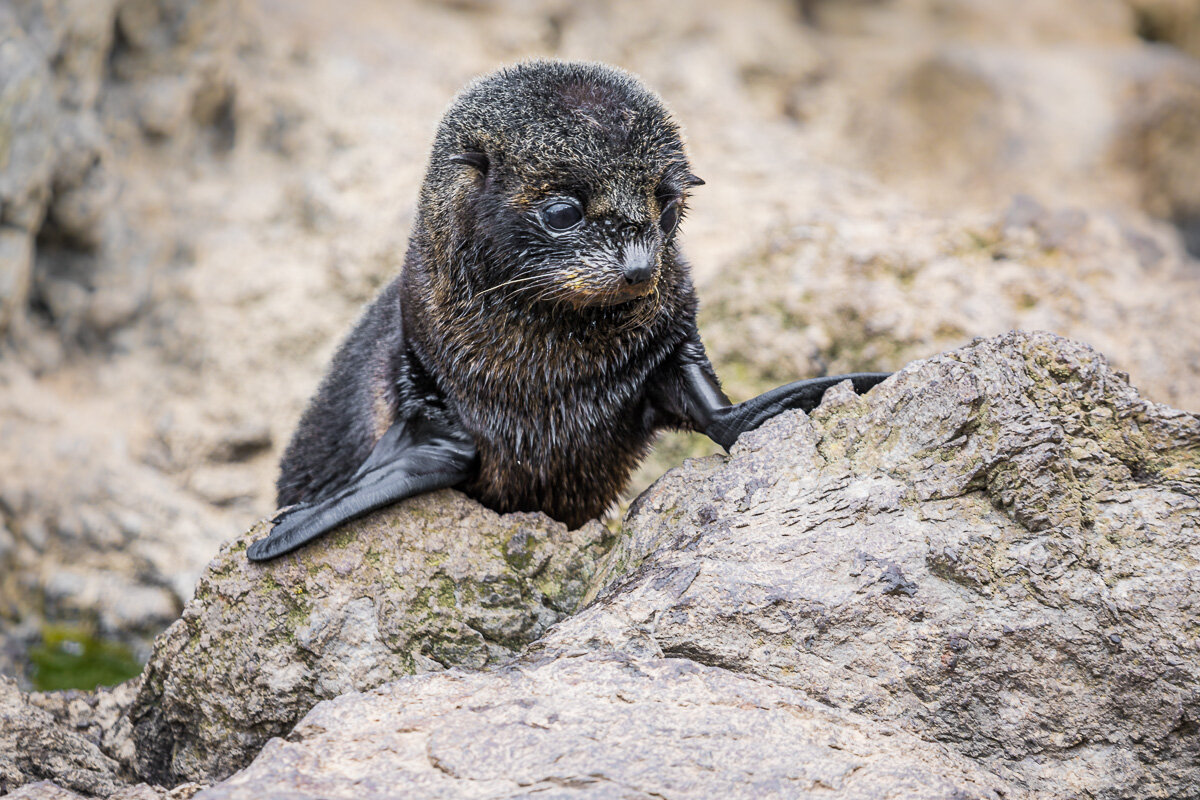In this close-up photograph, the central focus is a baby elephant seal. This adorable marine creature, possibly just a few days old, has sleek, dark fur speckled with hints of brown and yellow, lending it a freshly wetted appearance. The baby seal's striking black eyes, delicate little whiskers, and cute grayish-black nose stand out sharply against its fur. Its tiny black flippers, looking almost oil-slicked, are positioned on a large, well-lit sea rock that occupies the bottom right third of the image.

The baby seal, peering downward to the right, gives an impression of cautious exploration, perhaps indicating its newness to the world. The background features more out-of-focus rocks, enhancing the rocky seaside setting. A small patch of green vegetation is slightly visible in the bottom left, adding a touch of contrast. The overall composition and good lighting highlight the charming innocence and vulnerability of this young elephant seal as it navigates its rocky surroundings.